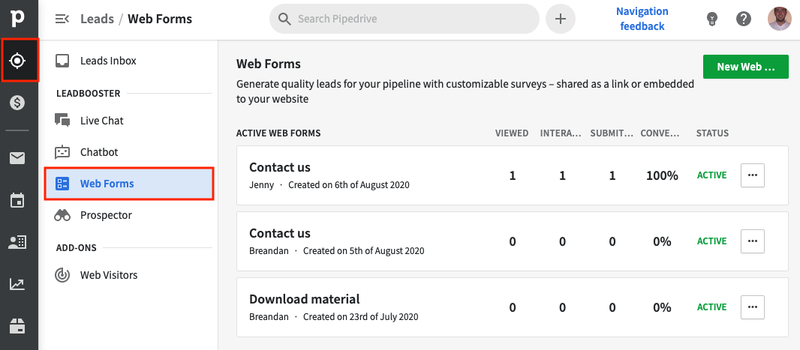The image captures a section of a web interface, presented with a clean, organized layout. On the far left of the image is a black vertical navigation bar featuring various option icons. Starting from the top, these icons are:

1. A white "P" in a black circle.
2. A compass or location icon, highlighted with a red square indicating selection.
3. A white circle containing a dollar sign.
4. A white envelope icon.
5. A calendar icon.
6. A silhouette of a person next to a square or building.
7. A line graph with an upward trend arrow.
8. An indistinct icon that appears to be either a file or a car door.

Adjacent to the left navigation bar, the main background is a clean mix of white and gray. A horizontal white bar at the top contains the text "Leeds - Web Forms" where "Web Forms" is in black. To its right is a gray search bar with a magnifying glass and the text "search pipe drive." Next to the search bar is a circle with a plus symbol, followed by a blue text link "navigation feedback." Further right, there are three more icons: a light bulb, a question mark within a gray circle, and a circle displaying an individual’s face.

Below the "Leeds - Web Forms" header, another white section lists several options, including:

1. Leads inbox
2. Lead booster
3. Live chat
4. Chat box
5. Web Forms (selected, highlighted in blue with a red outline)
6. Prospector
7. Add-ons (with the add-on "web visitors")

To the right side of the image, within the "Web Forms" section, it displays instructions and information: "Generate quality leads for your pipeline customizable survey shared as a link or embedded to your website." Below this message is a green button labeled "New Web."

Further down, under the "Active Web Forms" heading, the section lists columns of information categories: "Viewed," "Intro" (partially cut off), "Submit" (partially cut off), "Conv." (cut off indication of Conversion), and "Status." The data entries display three forms:

1. **First form:**
   - Title: "Contact Us, Jenny"
   - Created on: 6th August 2020
   - Viewed: 1
   - Intro: 1
   - Submit: 1
   - Conv.: 100%
   - Status: Active
   - Options: A white box with three horizontal dots

2. **Second form:**
   - Title: "Contact Us, Brendan"
   - Created on: 5th August 2020
   - Viewed: 0
   - Intro: 0
   - Submit: 0
   - Conv.: 0%
   - Status: Active
   - Options: A white box with three horizontal dots

3. **Third form:**
   - Title: "Download Material, Brendan"
   - Created on: 23rd July 2020
   - Viewed: 0
   - Intro: 0
   - Submit: 0
   - Conv.: 0%
   - Status: Active
   - Options: A white box with three horizontal dots

This detailed layout demonstrates a snapshot of a digital workspace, organized for managing and analyzing web forms and lead generation efficiently.